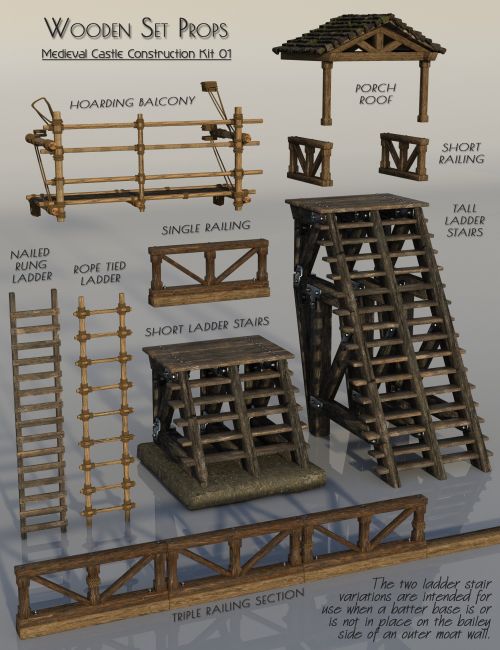The image is a detailed advertisement photograph of a wooden set titled "Wooden Set Props, Medieval Castle Construction Kit 01." The rectangular picture, taller than wide, showcases various wooden components against a background that grades from white to gray, becoming darker at the bottom. These components, all brown in color, include a hoarding balcony, a porch roof, short railings, a tall ladder stairs, a single railing, a rope-tied ladder, a nailed rung ladder, short ladder stairs, and a triple railing section. In the lower right-hand side, the image notes that the two ladder stair variations are intended for use when a batter base is or is not in place on the bailey side of the outer moat wall. The kit appears crafted for either children or miniature model enthusiasts, with each piece meticulously designed and photographed, possibly against a reflective surface that adds depth through shadows and subtle reflections.